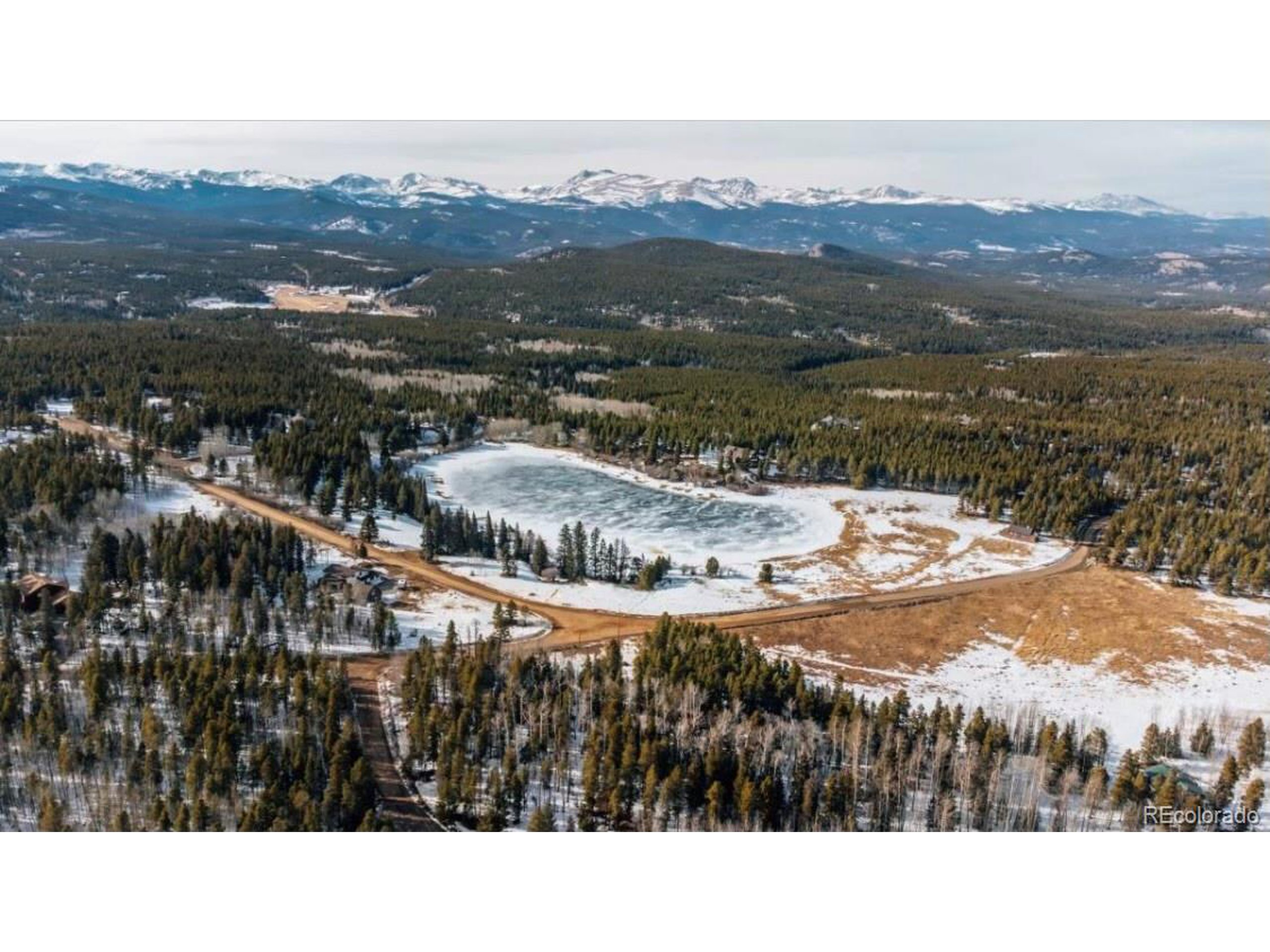This aerial photo captures a sweeping view of a forested landscape characterized by a kidney-shaped frozen lake at its center. The area is dotted with pine trees that feature the tall, narrow silhouettes typical of far northern or northwestern regions, reminiscent of tundra environments. The scene is intricately webbed by dirt roads that wind through the dense forest, providing paths that lead towards the icy lake. In the background, the terrain rises into partially snow-cleared hillsides, while the banks of the lake remain covered in snow. Far off in the distance, a range of snow-capped peaks majestically stretches across the horizon, under a light gray, cloud-covered sky. Situated possibly in regions like Montana or Utah, this picturesque outdoor nature scene conveys a cold but not wholly snow-blanketed landscape, marked by patches of green amidst the snowy expanse and large bluish-gray mountains overseeing the tranquil frozen lake.